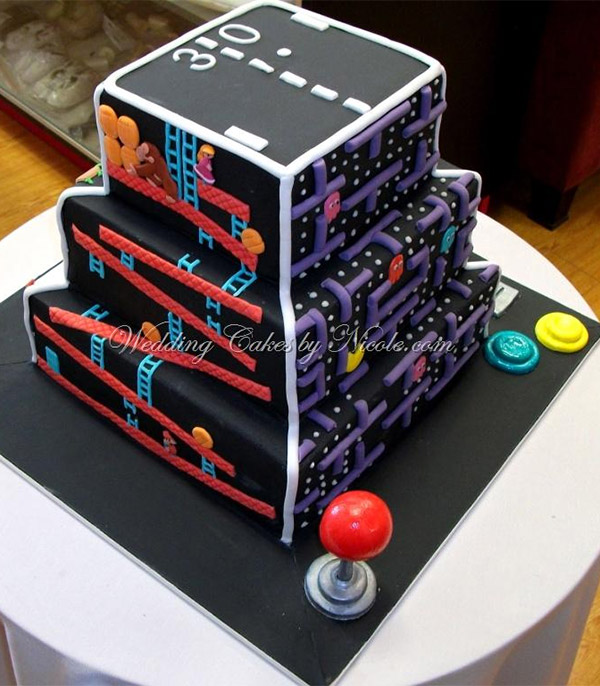This detailed description captures the key elements from each voice caption:

This image showcases an intricately designed, three-tiered cake that embodies a vintage video game theme, created by Wedding Cakes by Nicole.com. The cake is covered in black icing with white trimming, and each tier highlights a different classic video game. 

On the left side, there's a depiction of Donkey Kong, complete with the iconic ladder and princess rescue scene, crafted with a lot of fondant for a realistic, detailed look. On the front, which appears more to the right due to the angle of the photo, features Pac-Man chasing ghosts through a maze. The top of the cake portrays the retro game Pong, with a digital score of 3-0 divided by lines.

The cake is set upon a base designed to resemble an old-school arcade console, including a red joystick that resembles a Tootsie Pop and two fondant buttons – one yellow and one blue. The entire creation rests on a round table with a wooden floor, suggesting an indoor setting. The text "Wedding Cakes by Nicole.com" appears prominently on the cake, either as part of the design or added via photo editing. This elaborate piece acts as both a celebration of vintage gaming and a unique wedding cake.